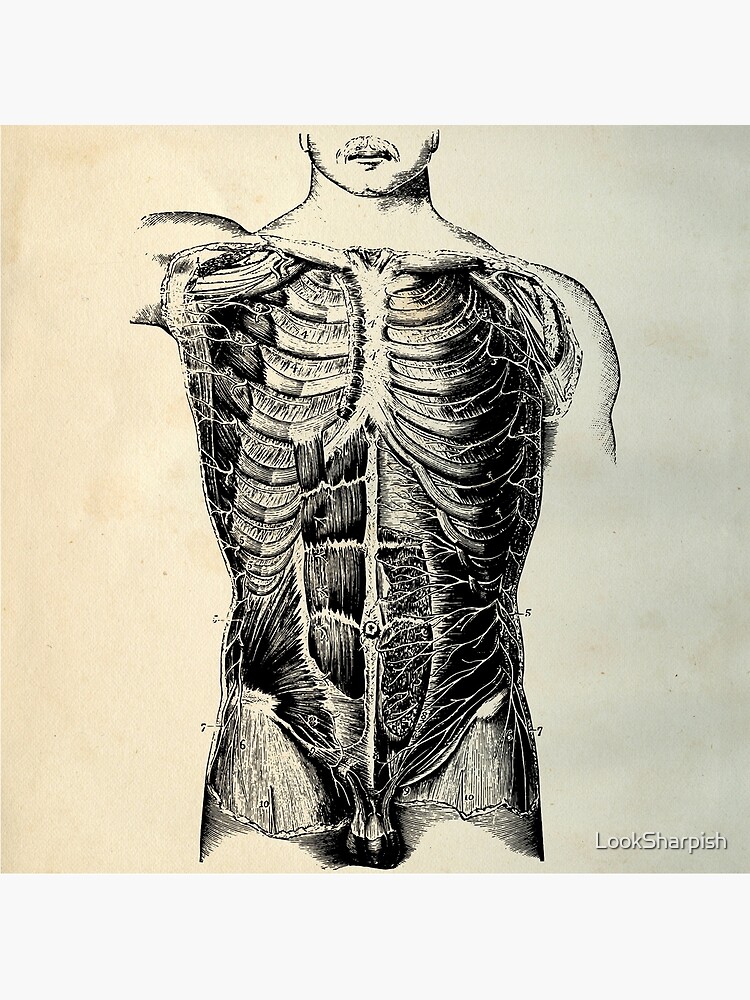This image features a highly detailed black and white sketch of a human torso, depicted in a vertically rectangular format with a thin gray border at the top. The central square image has contrasting colors with red on the left and blue on the right sides. There is a small amount of white text in the lower right corner, stating "look sharpish."

The drawing illustrates a man's torso from just below the nose, revealing a mustache and the bottom section of his face. The skin is intact from the neck upward and extending over the shoulders. However, from the neck down, the skin is removed to expose the underlying musculature and skeletal structure. The ribcage is prominently displayed, colored white with black stripes, drawn with pen or pencil for detail, and it spans from the chest down to the upper thighs. The stomach area is divided into three sections, showing intricate muscle striations in black. On the right side of the torso, the image reveals the nerves and veins that overlay the stomach muscles. Numerous lines point out various anatomical features, enhancing the diagram's instructional value.